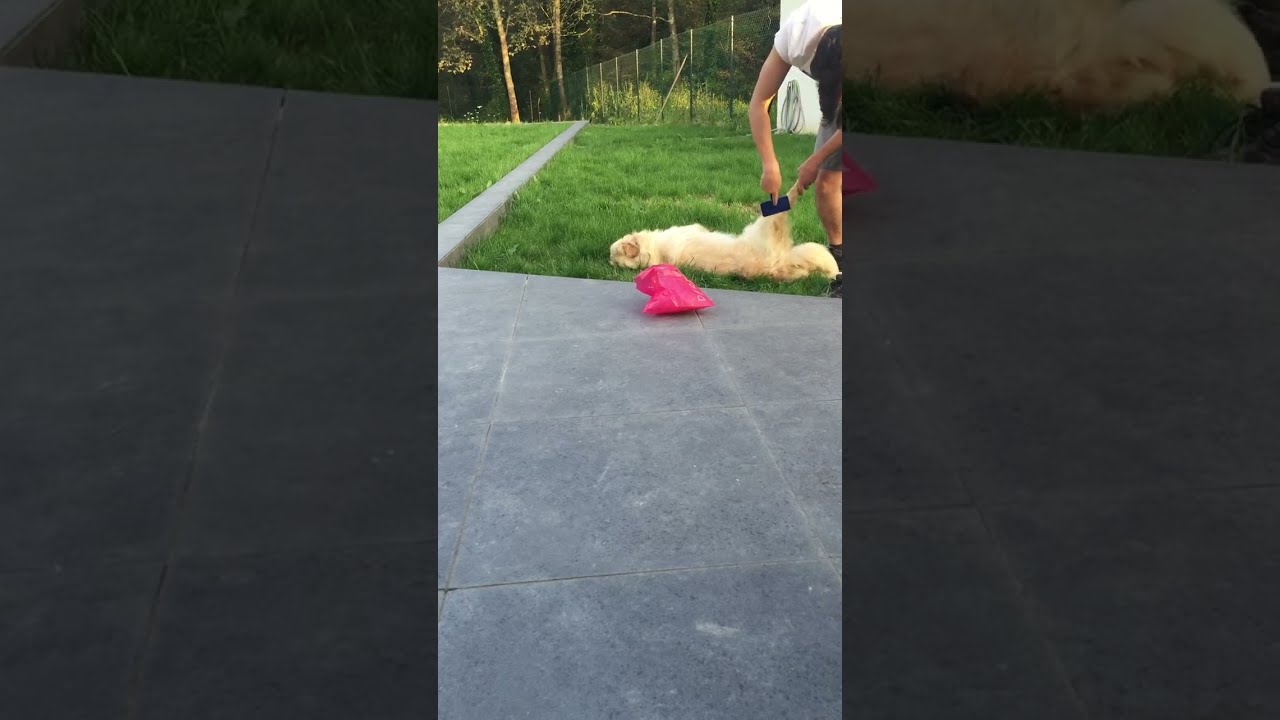The image is a photograph or a still from a video, framed as a horizontal rectangle with vertical black bars on the left and right sides. In the center third of the image, a dog is lying in the grass, facing slightly backward with one ear flopped over its face. The dog's body is oriented forward towards the background, with its right leg slightly raised and its tail straight down.

Beneath and around the dog, the ground is a mix of dark, blackish square tiles and patches of green grass. A small concrete path divides the grassy area, running straight towards the background. Adjacent to the dog, there is a red bag lying open.

In the background, a white building wall can be seen with a hose wrapped around it, alongside a tall fence that appears made of wire or barbed wire. Behind this fence, there are trees that complete the outdoor, daytime backyard setting of the image. The prominent colors include black, gray, white, green, and hints of magenta and brown.